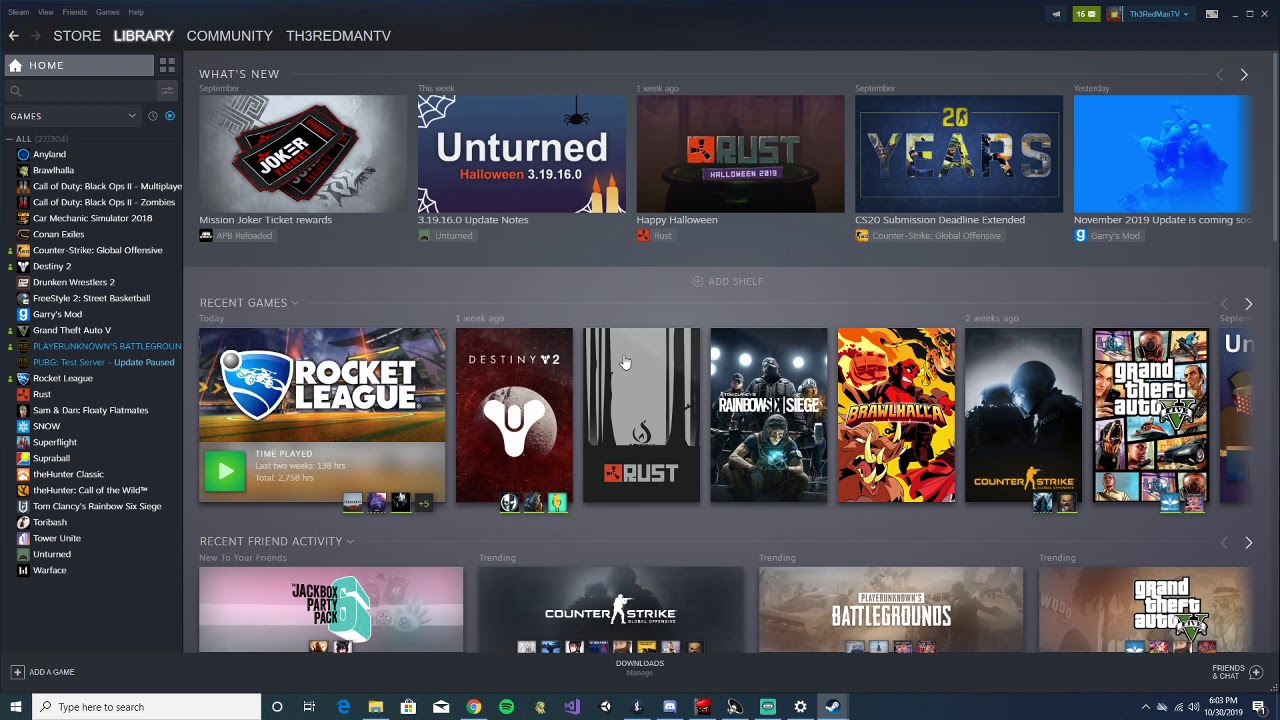This image is a screenshot of a gaming website displayed on a Windows computer. The webpage features a predominantly gray background and showcases a variety of video games by displaying their cover art. Visible game titles include "Grand Theft Auto," "Counter-Strike," "Rust," "Destiny 2," and "Rocket League." 

In the top left-hand corner of the page, there are four navigational options: Store, Library, Community, and Threads. At the bottom of the screenshot, the Windows taskbar is visible, featuring several program icons like Google Chrome, Spotify, and Internet Explorer. On the left side of the webpage, there is a lengthy list of approximately 30 games, providing a comprehensive selection for browsing.